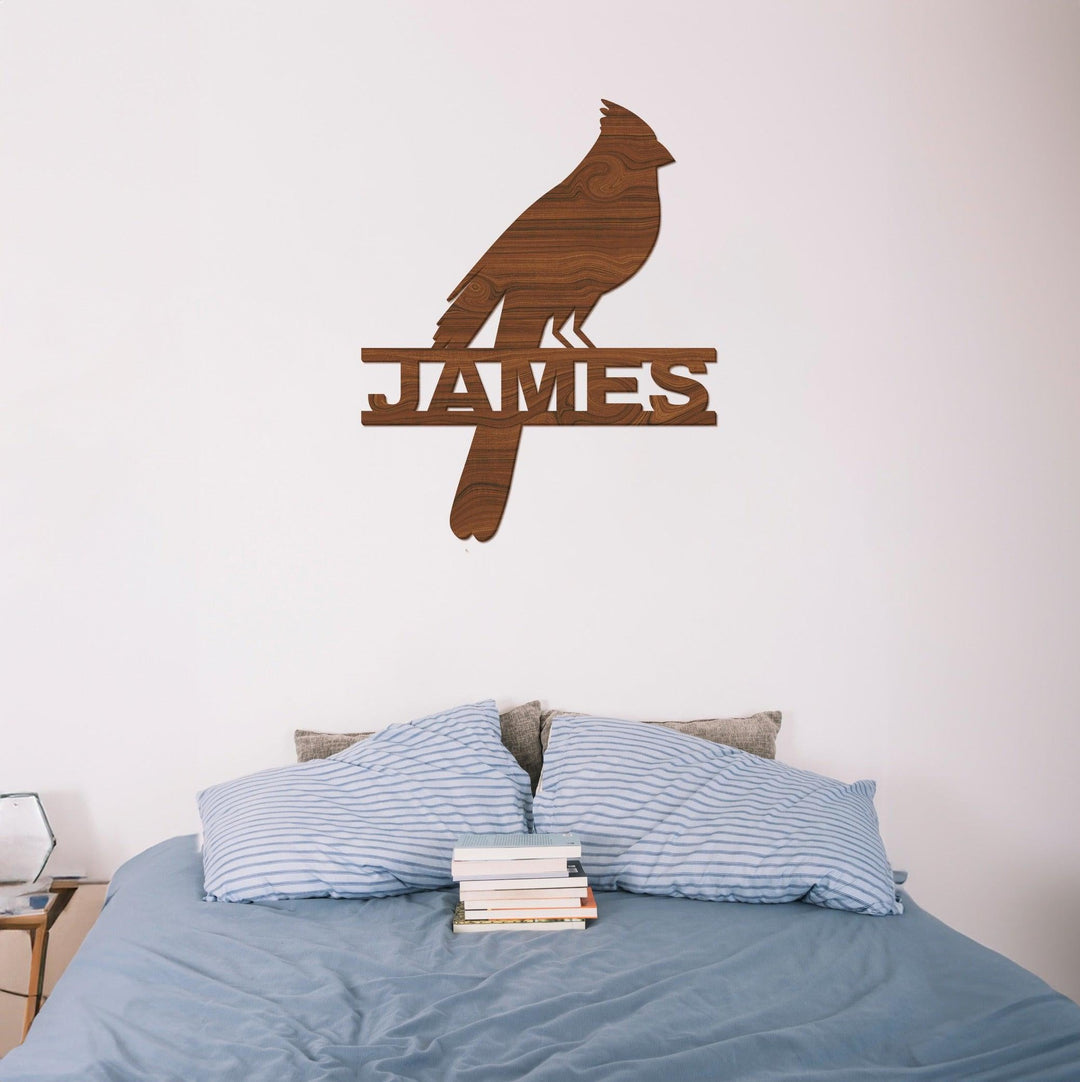This is a detailed interior shot of a bedroom with a light-colored wall that transitions to a slight pink hue in the top right corner. Mounted on the wall is a dark wooden design featuring a bird facing to the right. The bird is perched on a name sign that reads "James," with the name sandwiched between two surfaces and the bird's tail hanging below the letters. Below this artwork is a bed adorned with a blue comforter and blue striped standard pillows. Behind these are two smaller gray pillows. In front of the pillows sits a stack of books with the pages visible, not the spines. To the left of the bed, there is a small nightstand or a desk, possibly with an open display book lamp on top. The room's serene and slightly whimsical decor adds a personalized touch, making it a cozy and inviting space.